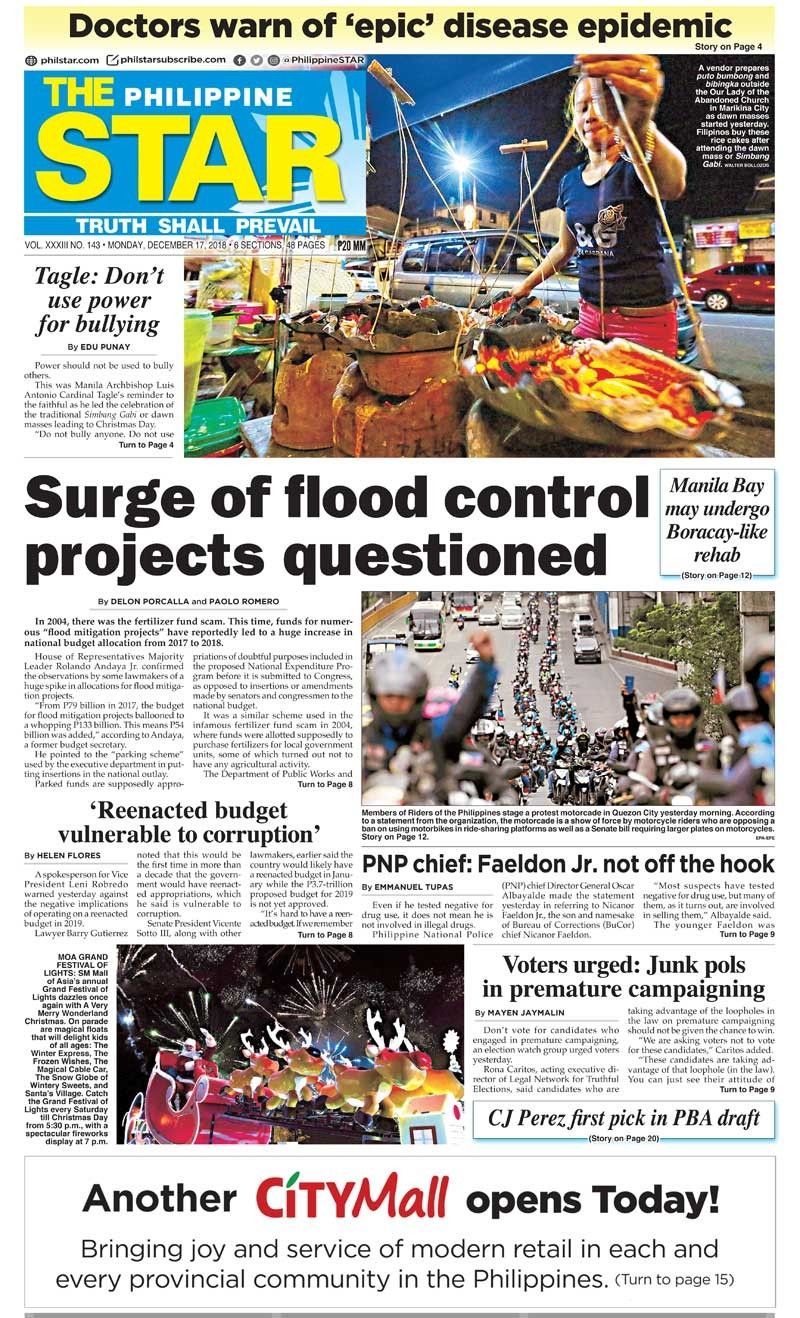Front Page of the Philippine Star: A Detailed Overview

The front page of the Philippine Star features a highly engaging and busy layout, particularly concentrated in the upper left-hand corner. The title "The Philippine Star" is prominently displayed at the top, with "The" and "Star" rendered in yellow, and "Philippine" in white, all set against a blue background. Directly below the masthead lies the newspaper's slogan: "Truth Shall Prevail."

Dominating the top section of this long sheet is a striking photograph of a female street food vendor, captured as she prepares food at night. Taken from behind her table, the image offers a bustling street view with cars in motion and various storefronts illuminating the background.

Adjacent to this primary image, the headline "Tagle: Don't Use Power for Bullying" grabs attention. Below the main photograph, another significant headline reads "Surge of Flood Control Projects Questioned."

Further down, the front page discusses several other topics of national interest:
- "Manila Bay May Undergo Boracay-Like Rehab"
- "A Show of Force by Motorcycle Riders," along with an image depicting a motorcade protest against the ban on motorcycles in ride-sharing platforms
- "Reenacted Budget Vulnerable to Corruption"
- "PNP Chief Albayalde Not Off the Hook"
- "Voters Urged to Junk Polls and Premature Campaigning"
- "CJ Perez First Pick in PBA Draft"

The only other image on the front page is a festive display: Santa Claus in a sleigh led by what appear to be balloon reindeer, set up in a public space, likely a mall, evoking the holiday spirit.

This vibrant and information-rich front page offers readers a deep dive into current events, public concerns, and festive cheer, encapsulating the diverse scope of the news that the Philippine Star delivers.